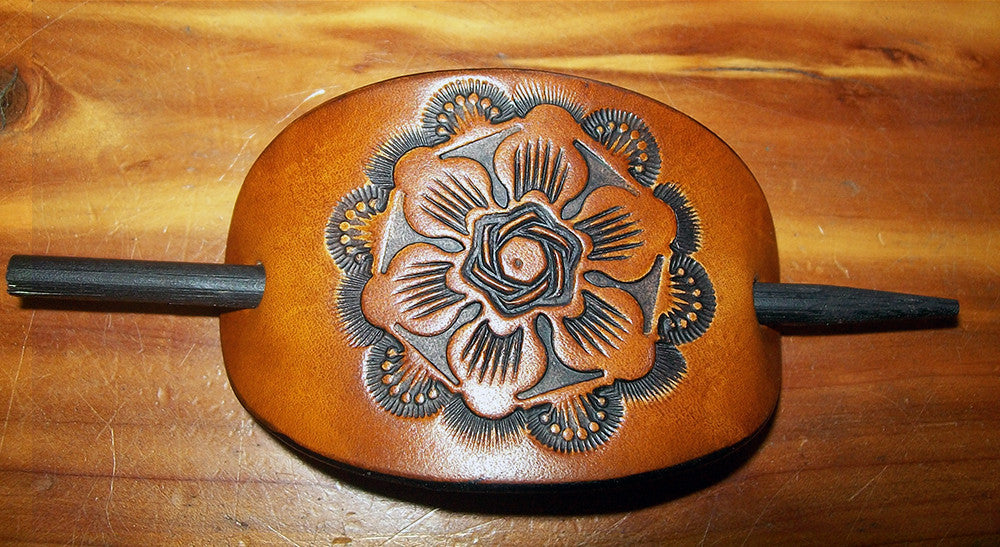This detailed photograph captures a handmade leather hair accessory displayed on a brown wooden table. The accessory itself is a brownish circular piece with an intricate design, featuring a large central flower stamped into the leather. This central floral design is surrounded by a honeycomb-shaped pattern, with additional geometric elements like upside-down triangles that contribute to its elaborate aesthetic. The outer edges of the accessory resemble doily-like arcs adorned with lines and dots. Through two holes on either side of this leather piece passes a black stick, flat on one end and narrower on the other, resembling a chopstick or pencil, used to secure the accessory in a hairstyle such as a ponytail. The overall color palette is muted, with various shades of brown and black predominating, creating a harmonious and eye-catching display that might be intended for an online listing, exemplifying both craftsmanship and functionality.